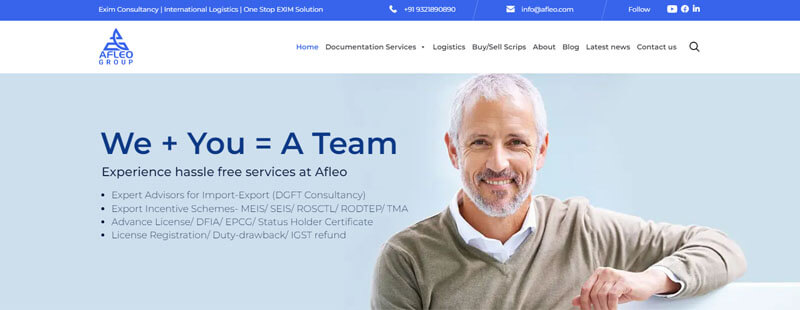This screen capture is from the AFLEO Group website, which appears to specialize in export advisory services. The image features an elderly white man with gray hair, a gray beard, and visible wrinkles, wearing a white collared shirt beneath a sweater. Next to the man, a message reads: "We + You = A Team." Beneath this slogan, it states, "Experience hassle-free services at AFLEO." AFLEO offers a range of services related to import-export, including export incentive schemes, advance licenses, DFIA, EPCG, status holder certificates, license registration, duty drawbacks, and IGST refunds.